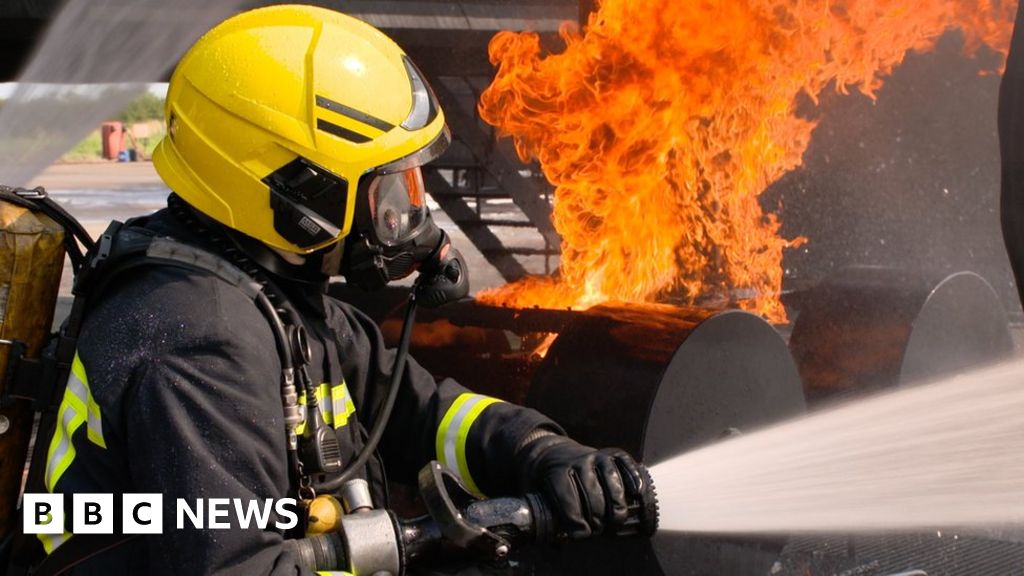In a scene captured from BBC News, a firefighter, clad in full gear, battles a raging blaze. The firefighter, presumed male, wears a black outfit adorned with yellow and white visibility stripes. A yellow helmet, featuring two black stripes and a clear visor, shields his head while an oxygen mask with a yellow tank is strapped to his back. Positioned to the left of the frame and facing sideways, he aims a powerful stream of water from a fully opened fire hose towards the inferno. The vivid orange flames illuminate the scene, with reflections visible in his visor. The environment is chaotic, possibly a basement area or parking zone, with nearby structures like wheels or tubes seemingly caught in the fire. In the background, steps are faintly visible amidst the smoke and flames. The bottom left corner of the image prominently displays the BBC News logo, emphasizing the gravity and immediacy of the situation.